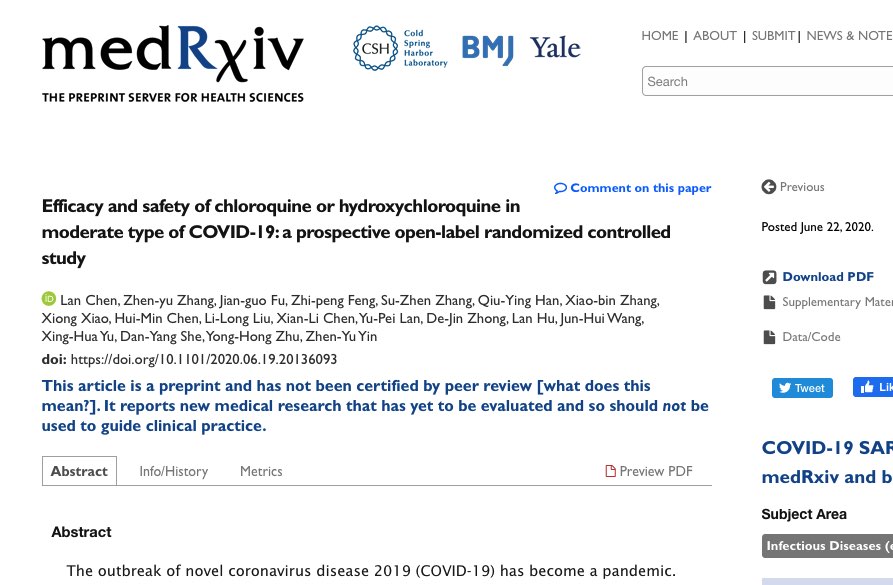At the top left corner, the text "M E D" appears in black writing followed by a capital letter "R" in a navy blue font. Next, a slightly slanted and lowered "X" in black font is visible, with "I V" in small, capital, black letters underneath it. To the right, a phrase in black reads, "the preprint server for health sciences."

To the right of this text, a circle is encircled by a blue chain link. Inside the circle, "C S H" is written in dark gray. To the right, in four separate lines of blue text, it reads "Cold Spring Harbor Laboratory."

Further to the right, in bold, blocky, navy blue lettering, "B M J" is written, with the end of the "J" pointed leftward and elongated. Adjacent to this is the Yale symbol, styled in a dark navy blue Times New Roman font.

To the right, a menu is visible with each option divided by a gray line. The menu options in light gray, from left to right, read: "Home," "About," "Submit," "News," and "Note."

Below this menu, a search field bordered in light gray displays the text "search" in light gray.

Below the search field, a headline in bold black reads, “Efficacy and Safety of Chloroquine or Hydroxychloroquine in Moderate Type of COVID-19: A Prospective Open-Label Randomized Control Study.”

Below the headline, a lime green circle with the white letters "I" and "D" occupies the center. The names of multiple authors appear underneath.

Below the author names, the text "D O I:" is in bold, black letters, followed by a URL in non-bold, black font.

Finally, a statement in bold navy blue font notes this is a preprint: "This article is a preprint and has not been certified by peer review." In brackets, "[What does this mean?]" follows in italicized font, along with an advisory note: "It reports new medical research that has yet to be evaluated and should not be used to guide clinical practice."